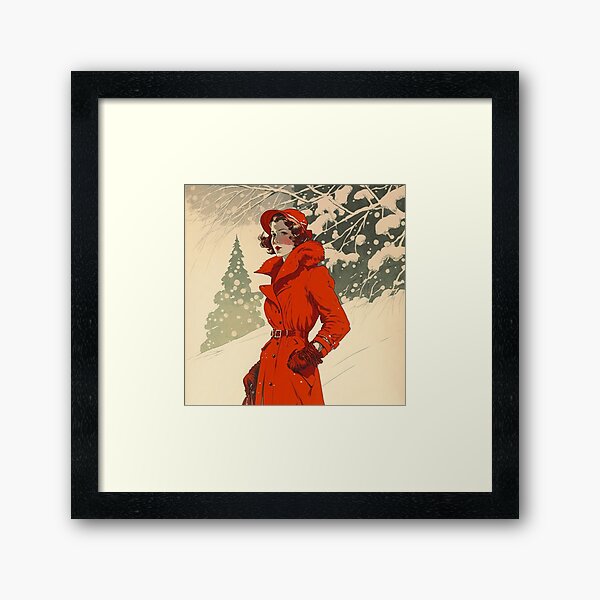The photograph showcases a large black-framed picture on a white wall, with a wide white mat inside the frame. This intricate artwork, seemingly a hand-drawn painting with a comic book style reminiscent of the 1960s, portrays a woman standing in a snowy landscape. Dressed in a red trench coat belted securely at the waist, accentuated with red fur around the collar, she accessorizes with matching red gloves and a broad-brimmed red hat. Her short, reddish-brown hair complements her red lipstick. The woman's left hand is in her pocket, while her right hand is elegantly positioned near her hip. The wintry background features a snowy hill and two snow-covered trees—a pine tree in the distance and another tree closer behind her—creating a nostalgic, vintage feel that echoes the style of the 1920s. She bears a striking resemblance to the iconic character Carmen Sandiego.